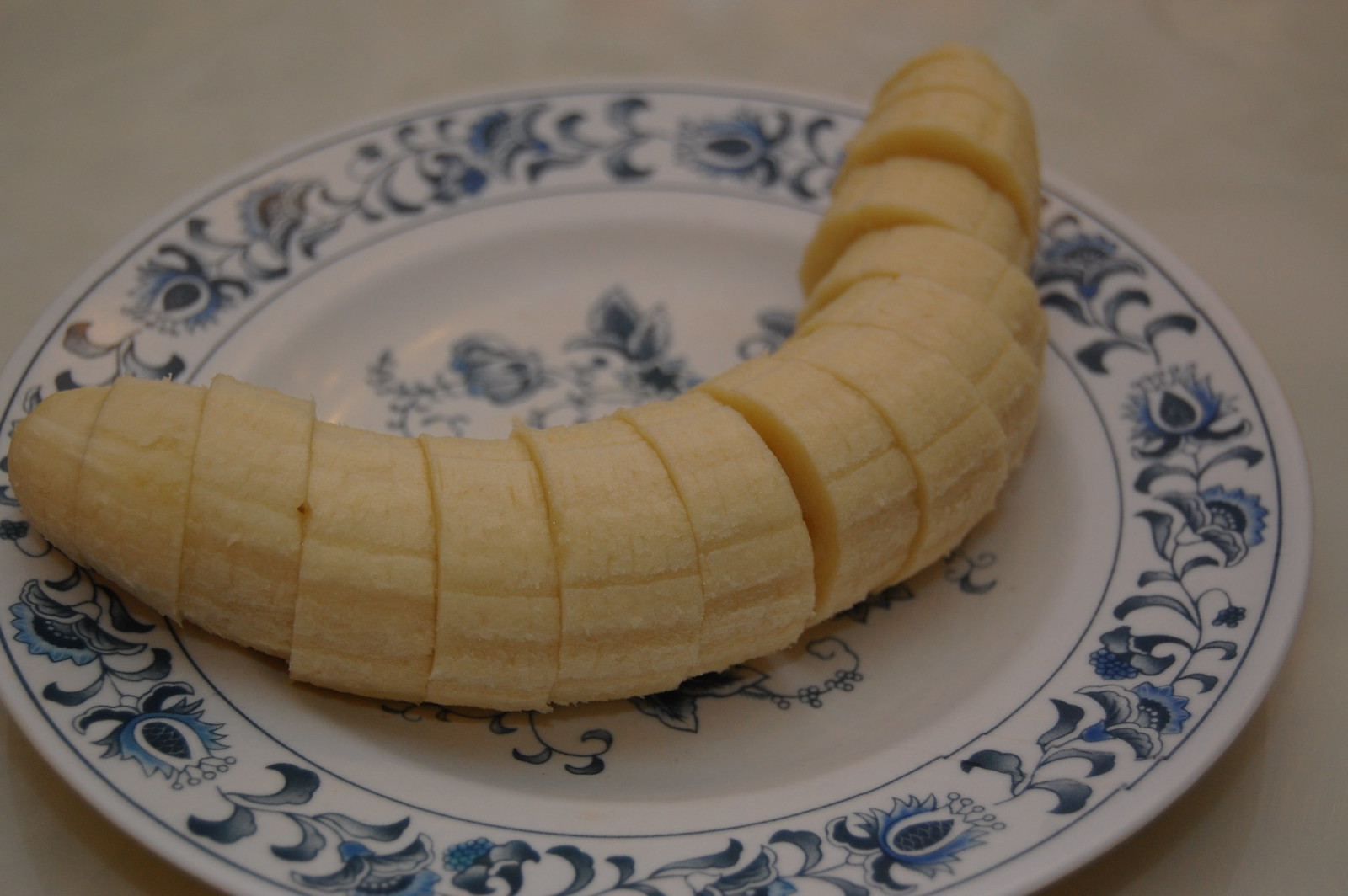In this close-up image, a small white plate with intricate blue floral patterns along its rim and a large central flower motif showcases an array of precisely fifteen banana slices. The arrangement of the banana slices fits perfectly within the confines of the plate, accentuating the decorative details of the dish. The off-white table beneath the plate is spotless, mirroring the cleanliness of the plate itself. This minimalistic yet aesthetically pleasing presentation focuses solely on the neatly sliced bananas and the detailed floral design of the plate, set against a simple, clean background.